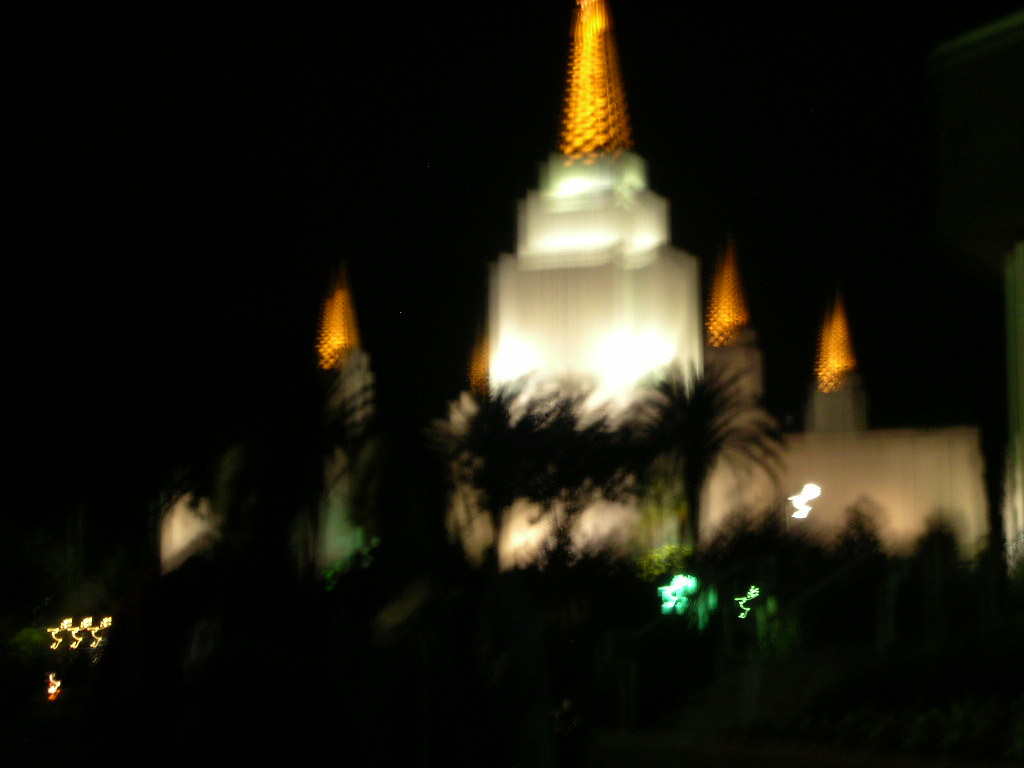The image depicts a very blurry and possibly jiggly photograph of a building at night, photographed with a slow shutter speed which results in a low-resolution, streaky effect. The scene appears to be set in a warm, tropical location, potentially Las Vegas, evidenced by the visible silhouette of at least four palm trees positioned among green bushes in the mid-ground. In the right section of the image, a tall grayish building with several distinct architectural features rises above the palm trees. This building is adorned with numerous bright yellow-orange, cone-shaped lights at the top, resembling flames. Additionally, scattered throughout this building are multiple similar yellow cones, contributing to the structure's illuminated appearance. The sky and foreground are pitch black, providing a stark contrast to the lit-up buildings. In the left part of the image, faint green neon stars are visible, although their source remains unclear. Overall, the chaotic blur and neon hues evoke a vibrant, possibly urban nightlife atmosphere.